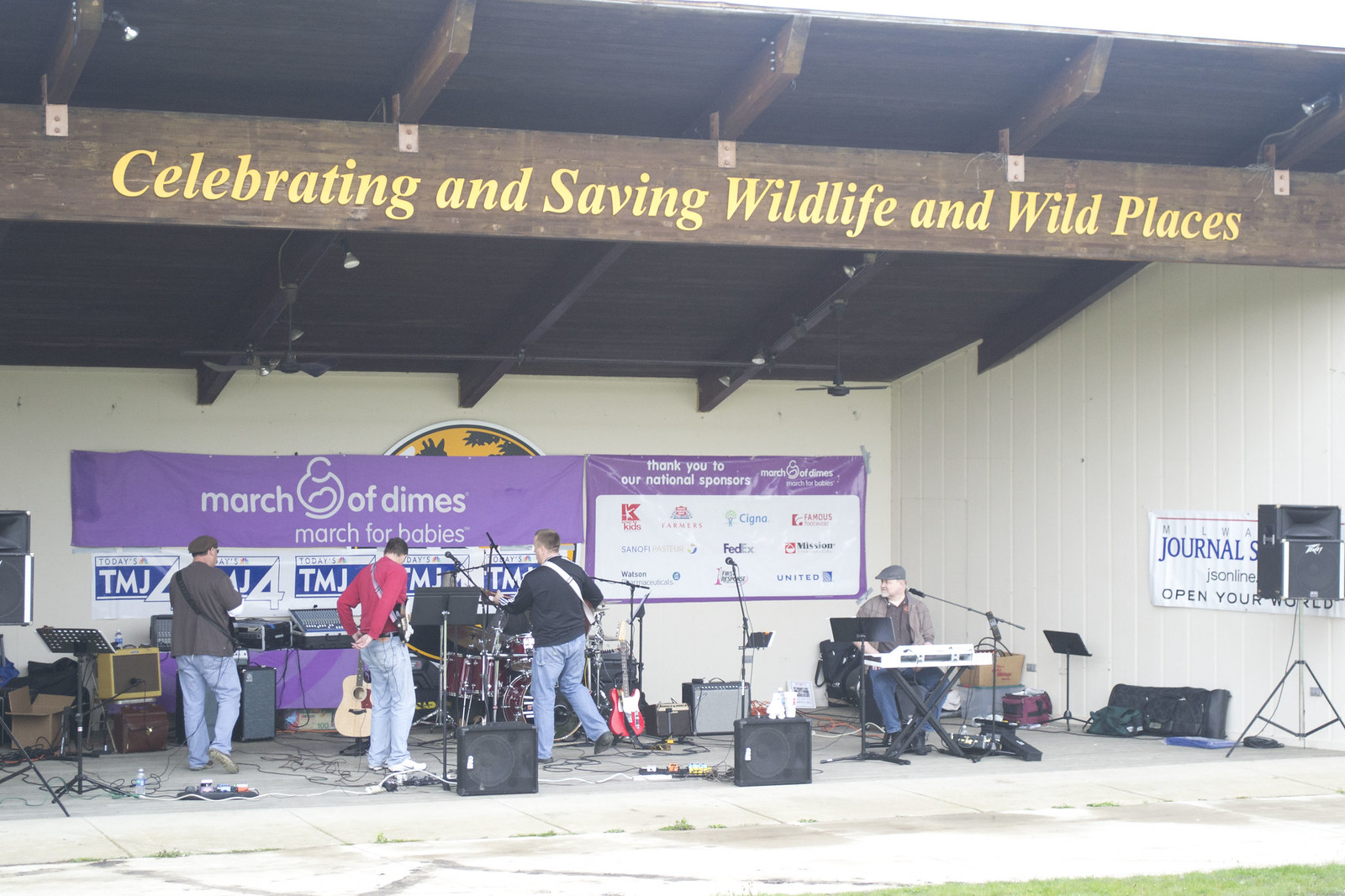The photograph depicts an outdoor bandshell stage, about a foot high, with a roof supported by a large brown wooden beam inscribed with "Celebrating and saving wildlife and wild places" in bold, italicized white font. The stage, a concrete platform with hints of grass in the foreground, features four men preparing for a performance: one seated at a white keyboard, and three others with guitars, their backs somewhat turned. The man in a red shirt has a shoulder strap, and another wears gray with a black strap, facing a drum set. The open-front structure has white walls and a gray and white floor. Microphones, speakers, wires, and various musical equipment are spread across the stage. In the backdrop, a prominent purple banner reads "March of Dimes, March for Babies," alongside another banner thanking national sponsors, including Cigna, FedEx, and United Airlines, with their logos prominently displayed.